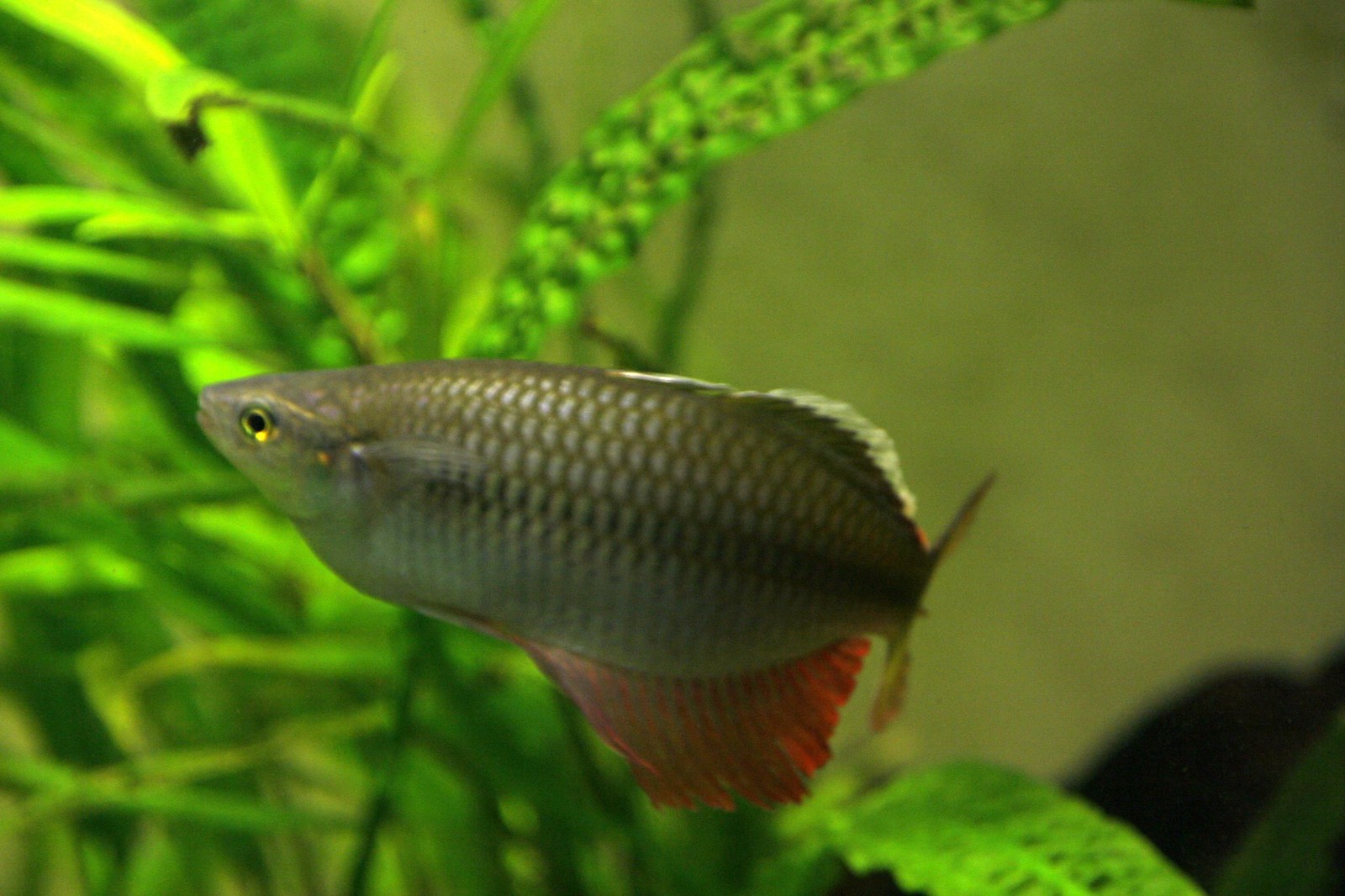This is a detailed close-up photograph of a small, oval-shaped betta fish situated in the center of a fish tank. The fish, characterized by its dark gray-brown scales and distinctive gold eyes, features a vibrant red bottom fin and a black and white top fin. The betta fish is facing to the left, with its tail to the right. Surrounding the fish, the background showcases lush green foliage, likely some sort of tall grass or seaweed, creating a rich aquatic environment. The water appears exceptionally clean, with the details of the fish and its immediate surroundings in sharp focus while the background remains slightly blurred. Additionally, there seems to be an indistinct red object, possibly a rock, at the bottom of the tank. The glass of the tank isn't visible, enhancing the natural feel of the scene. No text, name, date, or location information is present in the photograph.